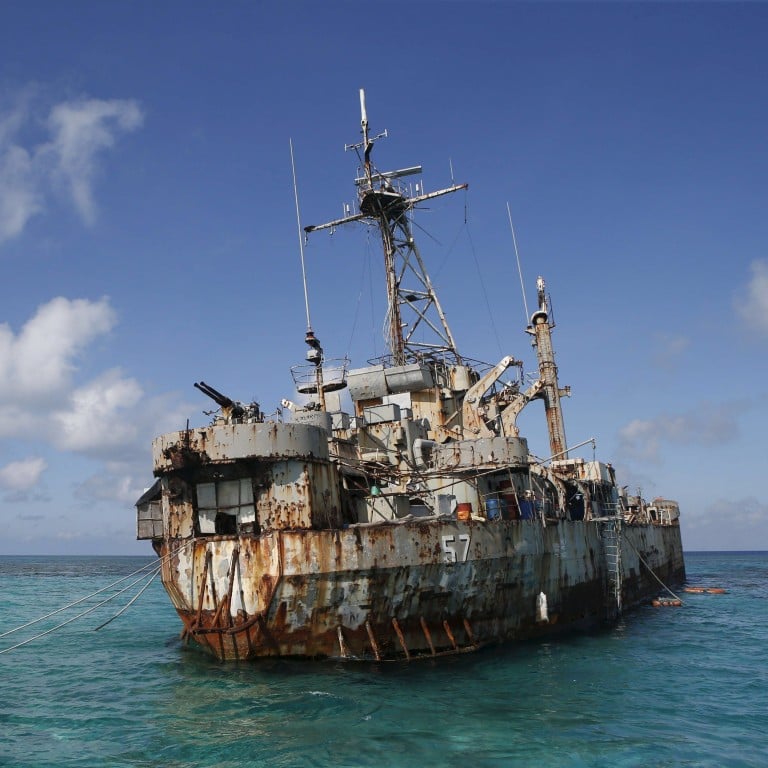The image depicts an old, worn-down warship floating in the ocean on a clear daytime. The ship, prominently rusted with a mostly gray hue, is centered in the frame, slightly tilted with its back end turned a bit to the right and its front end slightly left. The ship features the number "57" in white on its side. A large central mast and several ropes hang off the left side, hinting that it might be anchored. The vessel is visibly cluttered with various metal parts, compartments, and towers, giving it a crowded appearance. Notably, there's a round block of concrete near the front, supporting a gun turret with two barrels pointing upwards and to the left. The sky occupies the top two-thirds of the image, transitioning from a dark to light blue, adorned with wispy white clouds on the left and some gray clouds on the right. The darker blue ocean, replete with small wave ripples, spans the bottom third of the image.